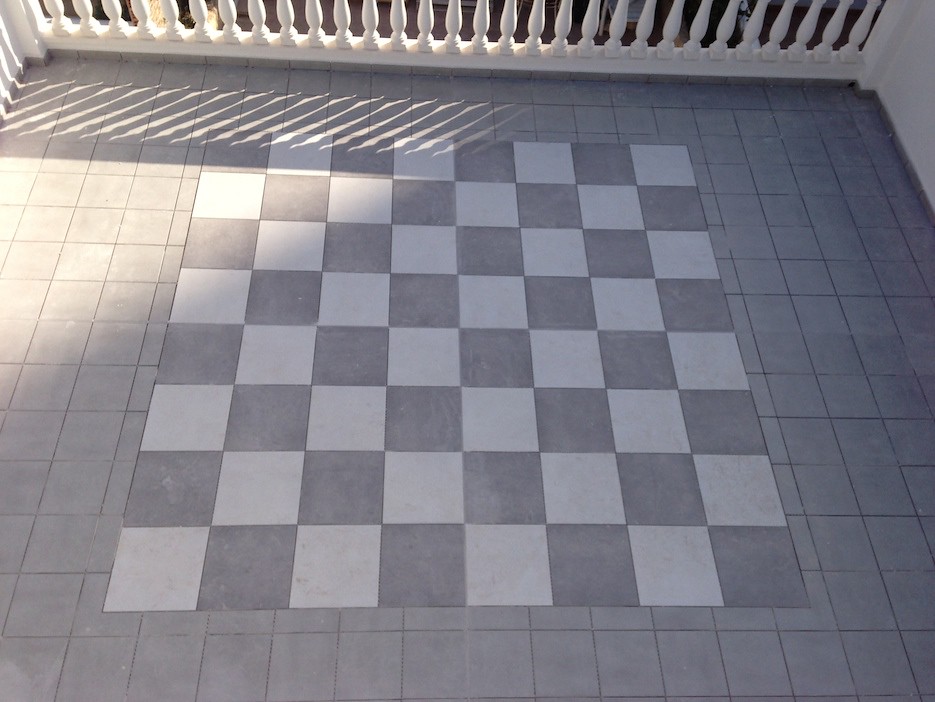This top-down photograph captures a spacious balcony, almost the size of a room, from a high vantage point. The balcony's floor is made up of small, smooth grey stone tiles, with a distinctive chessboard pattern in the middle, consisting of alternating larger grey and white squares. This checkerboard area is devoid of chess pieces but stands out prominently against the plain grey tiles that form the wide border around it. The balcony is enclosed by a white railing, or balustrade, designed to prevent falls, suggesting it's part of a multi-story house, likely above the first or second floor. The sun, in an early morning position, casts slatted shadows through the railing onto the balcony floor, adding a dramatic play of light and shadows to the scene. The two sides of the balcony feature solid white walls, framing the elegant outdoor space.